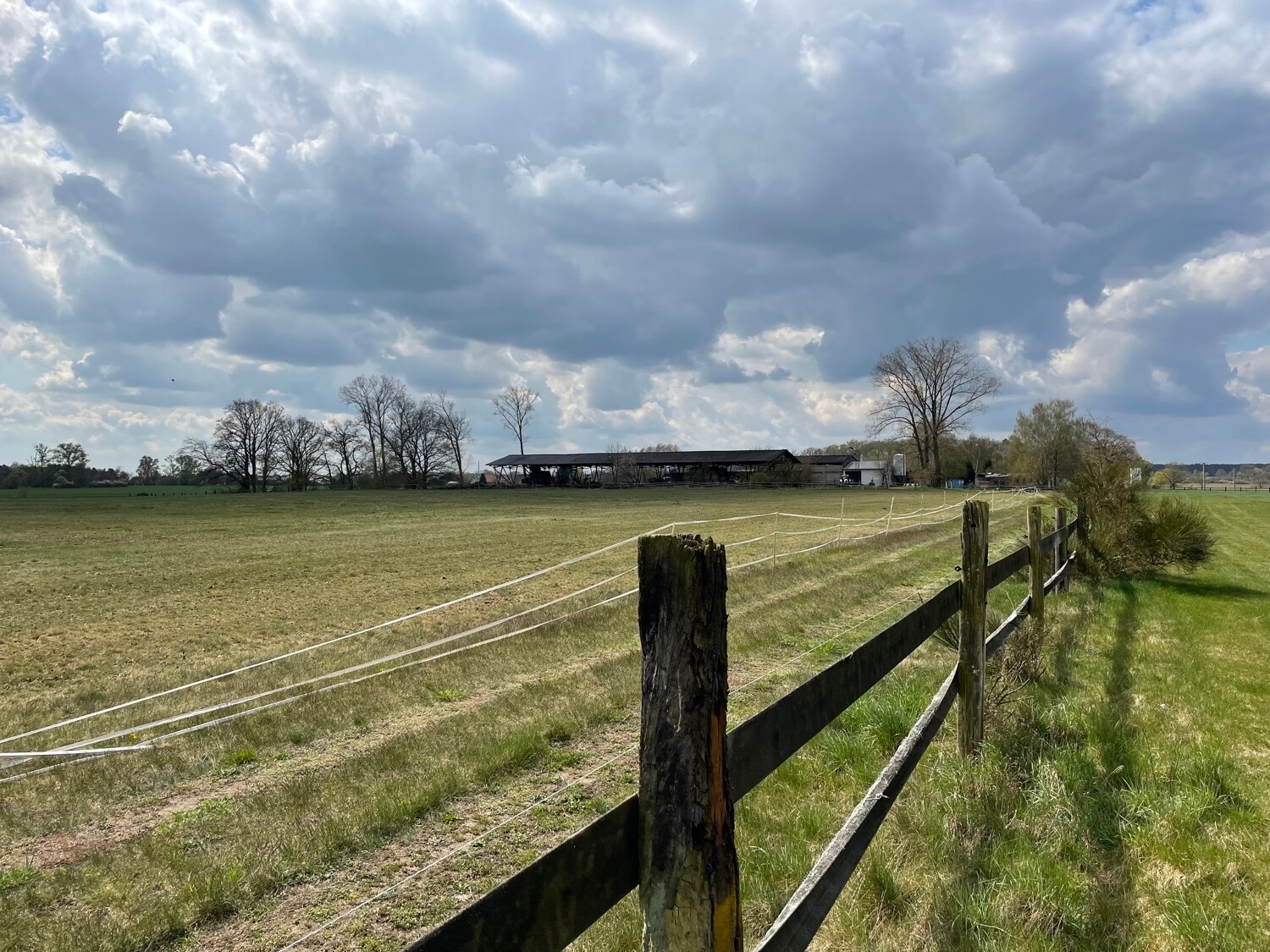This is an outdoor daytime photograph depicting a serene and expansive rural scene. Dominating the foreground is an old, slightly worn wooden fence that begins from the bottom center of the image and extends towards the right. To the right of the fence is a lush, untouched green field, contrasting with a more trodden, less vibrant field to the left that suggests frequent passage or light agricultural activity. This latter field features a faint white line and what appears to be a path made by repeated travel. The background showcases a rustic farm setting, with a barn and a house nestled among several trees, some healthy and full, others appearing bare with thin leaves. Numerous fluffy, dark clouds fill the upper half of the scene, hinting at an impending rain. The overall impression is one of tranquil rural life, with vast open spaces and a mix of untouched and cultivated land, surrounded by an undisturbed natural environment.